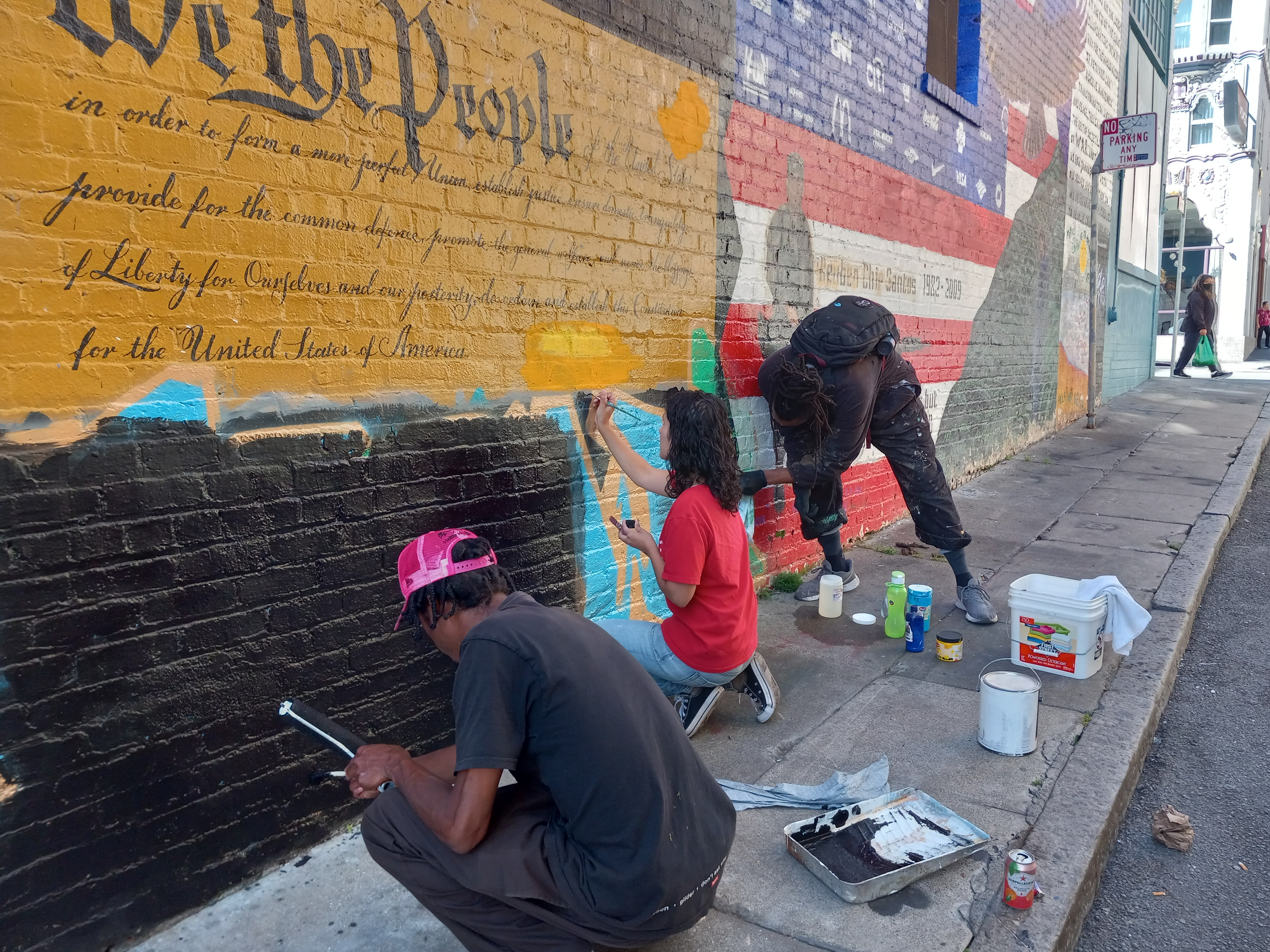The image depicts a vibrant scene on a city sidewalk where three individuals are engaged in painting a mural. Two are African American men dressed in black clothing, with one donning a striking hot pink baseball cap, and the third is a Caucasian woman with brown hair, wearing a red shirt and blue jeans. They are surrounded by paint supplies scattered on the ground as they work on the mural.

The mural itself is a detailed and multifaceted artwork. Dominating the scene are elements of the American flag interspersed with various dates and names that appear to honor fallen soldiers. One such name is "Ruben Chisantos, 1982-2009," suggesting a memorial aspect to the piece. In the upper right section of the flag, various corporate logos such as those of Citi, McDonald's, and Nike can be identified among an array of less discernible symbols.

Towards the left side of the mural, the opening phrases of the preamble to the United States Constitution, "We the People, in order to form a more perfect Union, establish...", are prominently displayed, adding a patriotic and foundational element to the artwork.

It is unclear whether the artists are creating this mural from scratch, restoring and brightening its colors, or covering up a previous piece of art. The mural's rich symbolism and the industrious activity surrounding it add layers of meaning and community engagement to the urban setting.